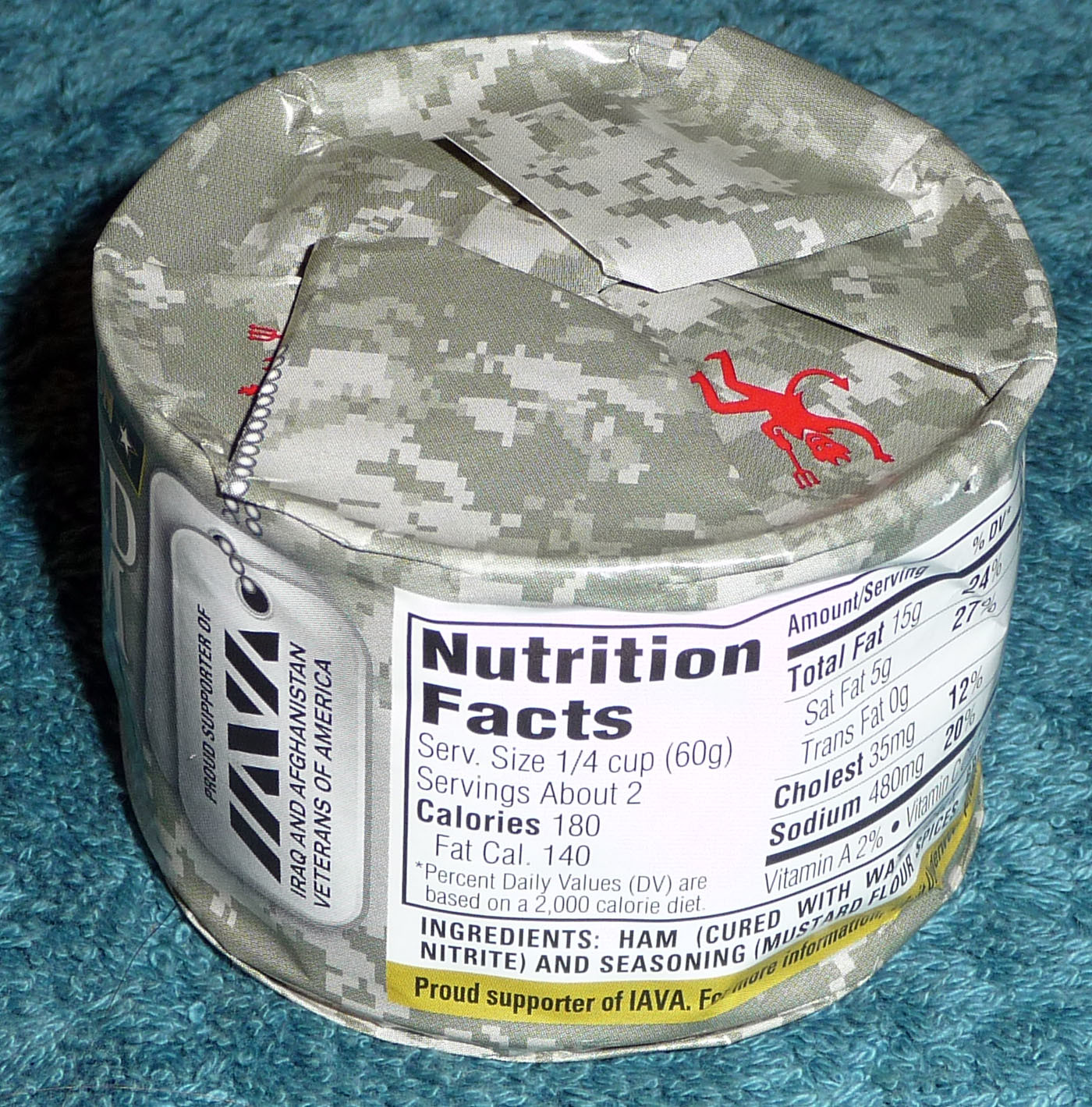This is a detailed photograph of a can of deviled ham, characterized by its distinctive camouflage-style paper wrapping. Prominently featured on the label is a red devil figure with one arm raised and holding a pitchfork, his curly tail ending in an up-pointing arrowhead. The label also includes a light gray image of two dog tags and a gold band bearing inscriptions that read, "Proud Supporter of Iraq and Afghanistan Veterans of America" and "Proud Supporter of IAVA." 

Nutritional information is provided on a white section of the label, indicating a serving size of 1/4 cup (60 grams) with roughly two servings per can, totaling 120 grams. Each serving contains 180 calories, with 140 calories from fat, including 15 grams of total fat, 5 grams of saturated fat, no trans fat, and 35 milligrams of cholesterol. The sodium content is listed at 480 milligrams, and it provides 2% of the daily value for vitamin A. 

The ingredients listed include ham cured with water, spices, and seasoning, although the complete list is partially obscured. Overall, the image conveys a sense of support for veterans, with the camo design and military associations suggested by the printed details on the can.